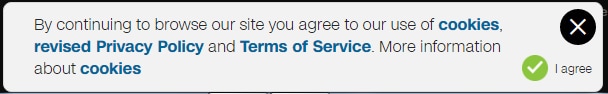Displayed prominently on many websites, this notice urges users to acknowledge and consent to the site's use of cookies and adherence to revised policies. The notice itself is bordered in black with a gray square at its center. Inside this square, the message is inscribed in black letters: "By continuing to browse our site, you agree to our use of cookies, revised privacy policy, and terms of service. More information about cookies." 

Key terms such as "cookies," "revised privacy policy," "terms of service," and the second instance of "cookies" are highlighted in blue, indicating they are clickable links for further information. 

To the right of this text, a white "X" is set within a black circular background, offering an option to close the notice. Below it is a green button embedded with a white check mark, smaller in size than the black circle, with the phrase "I agree" beside it. This button confirms the user's acceptance of browsing the site under the specified terms, including the use of cookies and adherence to the updated privacy policy and terms of service.